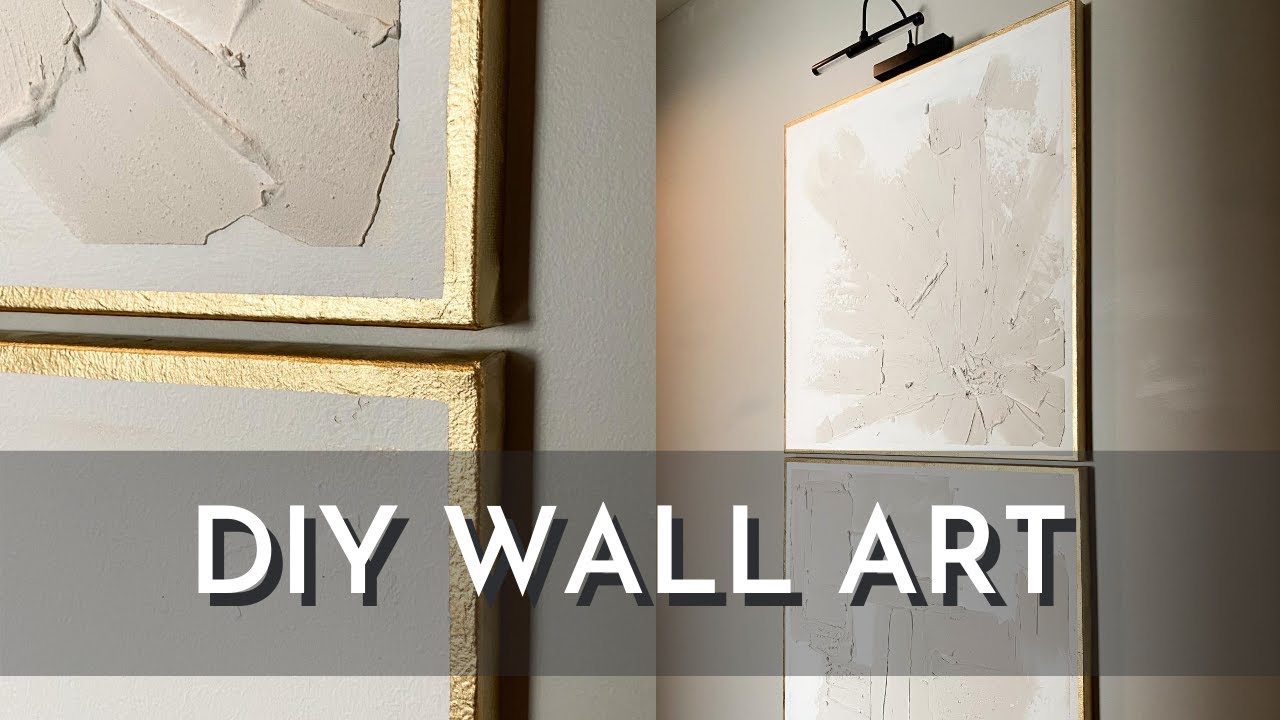The image appears to be an advertisement for DIY wall art displayed against a uniform gray background. There are three distinct pieces of wall art, each partially visible. The first piece shows only its bottom right corner, the second reveals its top right corner, and the third, almost fully visible but with the bottom cut off, is illuminated by an overhead lamp. The frames are accented with slender, gold-painted edges that blend seamlessly with the canvas, creating a modern, minimalist aesthetic. The artworks themselves feature various abstract compositions in shades of white and gray, appearing as indistinct blobs. In the bottom section of the image, a gray bar features bold, white text reading "DIY wall art," emphasizing the do-it-yourself nature of the pieces.